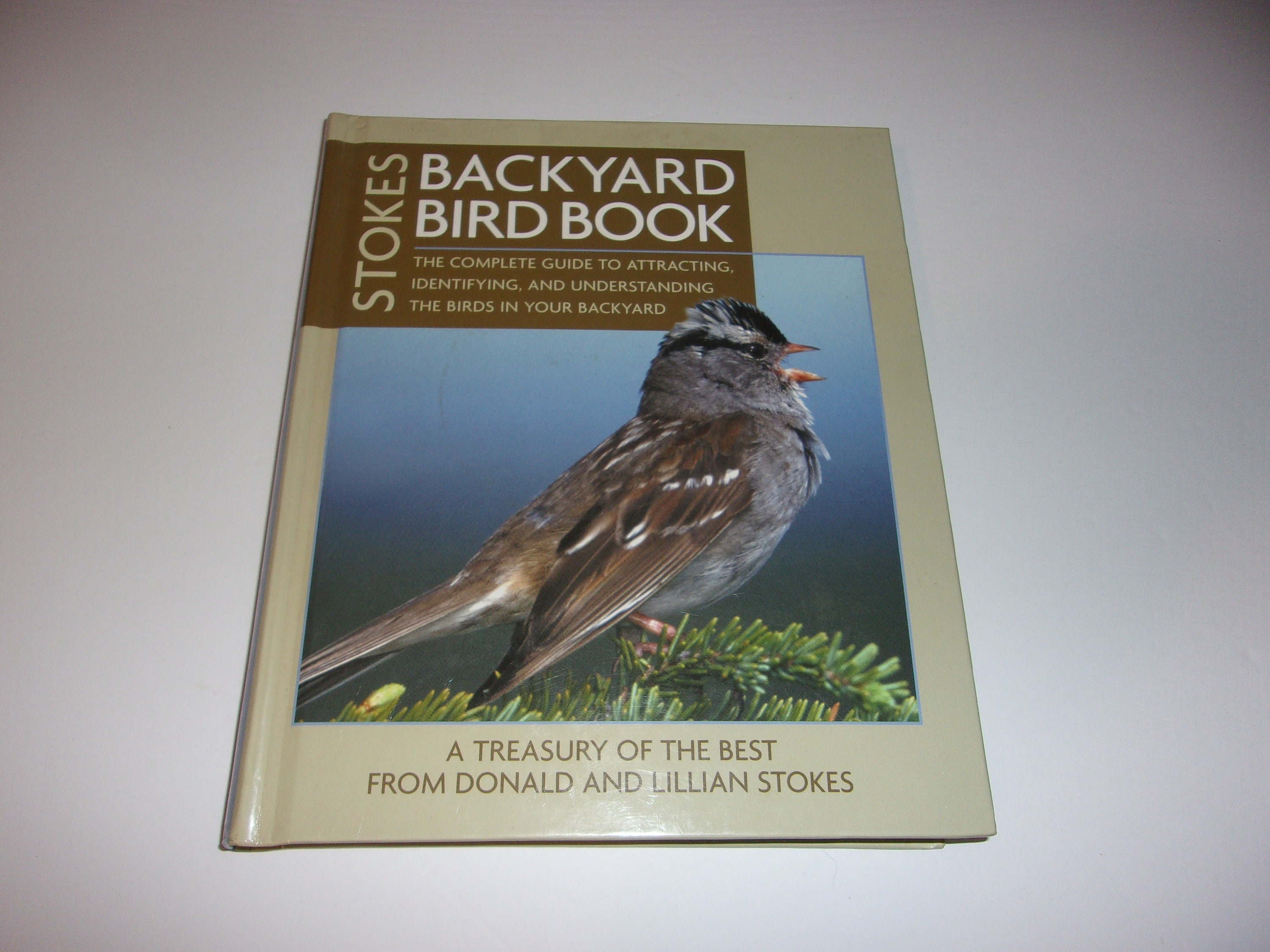The rectangular photograph, approximately six inches wide and four inches tall, depicts a thin hardback book laying on a light gray surface, though it's unclear if the surface is a table or countertop. The book's main color is a light tan. Its cover features a brown rectangular box with white print, positioned from the upper left-hand corner extending two-thirds to the right and down by about an inch. This box bears the title "Backyard Bird Book" in white print. To the left of this box, in tan text, it reads "Stokes," with the subtitle underneath stating, "The Complete Guide to Attracting, Identifying, and Understanding the Birds in Your Backyard."

Below the text, the majority of the cover is dominated by an image of a bird standing on a pine branch with a background that transitions from light blue at the top to darker blue at the bottom. The bird is facing to the right, its beak is orange, with a gray head featuring a black mohawk-like streak running down the center, and a black line extending from its eye. The bird's chest is gray, while its back, wings, and tail are brown. At the bottom of the cover, in brown print, it states, "A Treasury of the Best from Donald and Lillian Stokes." The book is positioned such that the bottom is closer to the viewer and the cover appears slightly tilted, causing some distortion in the perspective.